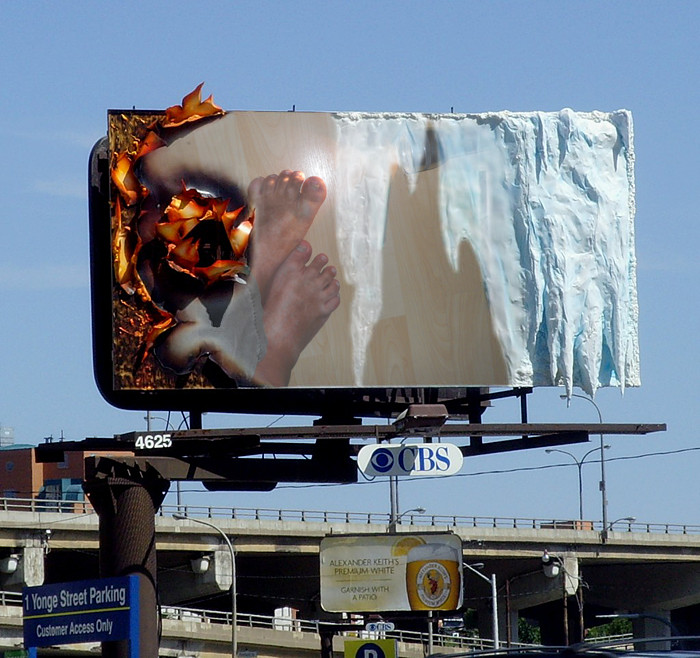The image prominently features a rectangular billboard, centrally located, that dramatically blends elements of fire and ice. The right side of the billboard is encrusted in ice, with crystalline spikes jutting outward, giving it a lifelike, three-dimensional appearance. In stark contrast, the left side is engulfed in flames, with charred, orange edges and a large ball of fire invading from the left-hand edge towards the center, where the image of a pair of feet is displayed. The background provides additional context, showcasing a blue sky and a typical American highway scene with an array of infrastructure details including bridges, signage, and a bronze metal stand supporting the billboard. Visible deeper in the background are additional billboards, one of which advertises Alexander Keith’s Premium White Garnish with a Patio, and another blue sign indicating "One Yonge Street Parking, customer access only." The confluence of fire and ice on the billboard juxtaposes scorching heat with frozen serenity, creating a visually striking and captivating image.